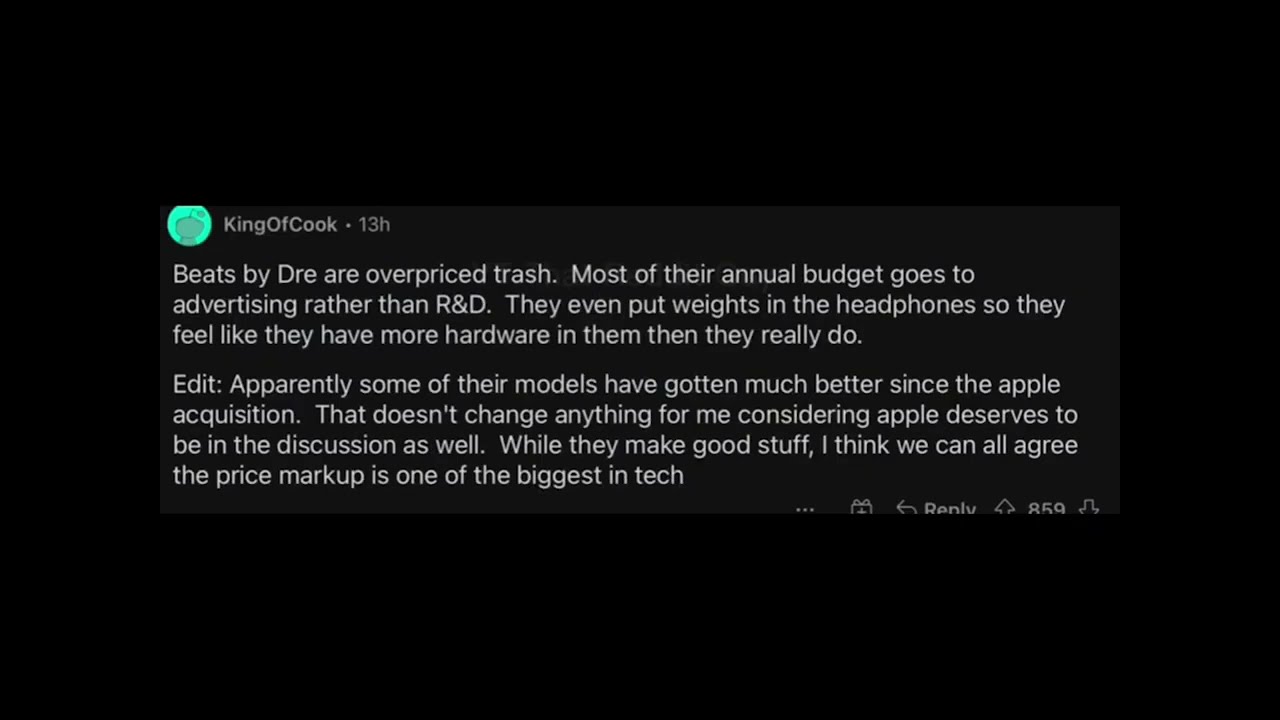The image features a Reddit post by the user "King of Cook," identifiable by a lime green avatar depicting the Reddit mascot. The post, surrounded by a black border and displayed in white text on a dark gray background, was made 13 hours ago, as indicated by the "13H" timestamp. In the review, King of Cook criticizes Beats by Dre headphones, calling them "overpriced trash" and alleging that most of the company's budget is spent on advertising instead of R&D. The user claims that the headphones even contain weights to create a false impression of substantial hardware. Despite acknowledging that some models have improved since Apple's acquisition, the user insists that Apple's significant price markup remains a critical issue. The sentiment of dissatisfaction is underscored by the review's 859 upvotes.